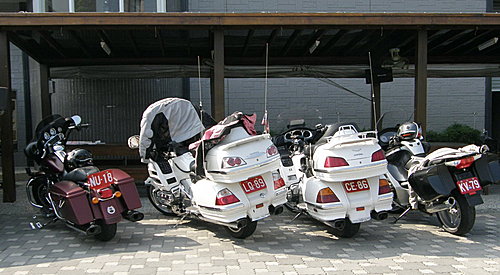This photograph, taken on a sunny day, showcases four motorcycles neatly lined up in a carport area paved with square gray bricks in varying shades. In the background, there is a dark brown carport structure with posts supporting it, casting shadows over the motorcycles and a white wall behind it.

From left to right, the motorcycles are as follows:

1. The first motorcycle is a dark burgundy, almost maroon color with matching hard saddlebags. It features a windshield, a black seat, and a red license plate displaying "NU-18." A helmet rests on its seat.

2. The second motorcycle is large and white, equipped with a windshield and a cover over the handlebars. It has substantial rear baggage compartments and red tail lamps. Its red license plate reads "LQ-89."

3. The third motorcycle is also white and resembles the second one, but it lacks the handlebar cover. It has similar hard bags and rear tail lamps, with a red license plate showing "CE-86."

4. The fourth and smallest motorcycle is black and silver. It has black saddlebags, a windshield, and a silver helmet positioned towards its front. Its red license plate is marked "KY-79."

The motorcycles evoke a mix of classical and modern aesthetics, particularly highlighted by the traditional design of the three on the left and the contemporary look of the one on the far right. The overall setting, with the neat alignment of the motorcycles and the structured paving, adds to the organized and somewhat serene outdoor scene.